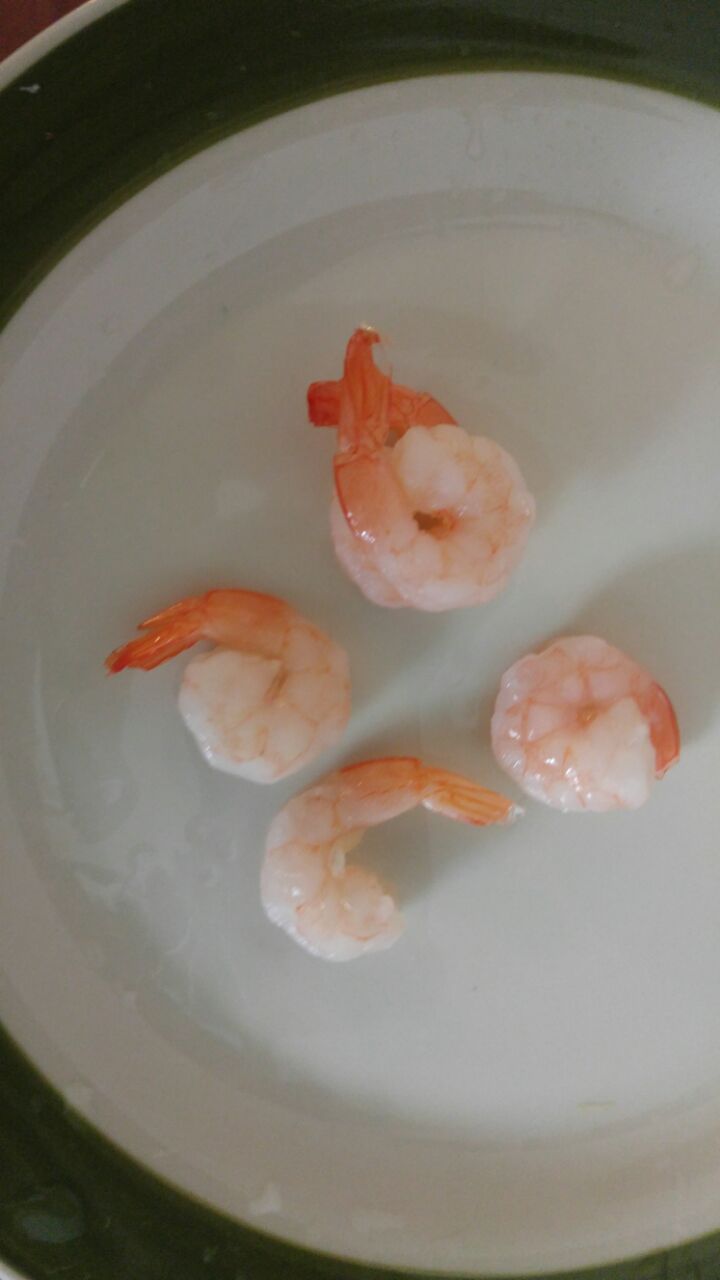The image depicts a white plate with a dark green rim, set against a black background. The plate features four cooked shrimp in various degrees of curl, ranging from slightly curled to tightly balled up. The shrimp, pinkish-white from cooking, still have their reddish-pink tails on. The arrangement makes the shrimp appear as though they are performing somersaults. The plate is devoid of any text or signatures, and the interior setting casts a noticeable shadow on the white surface.